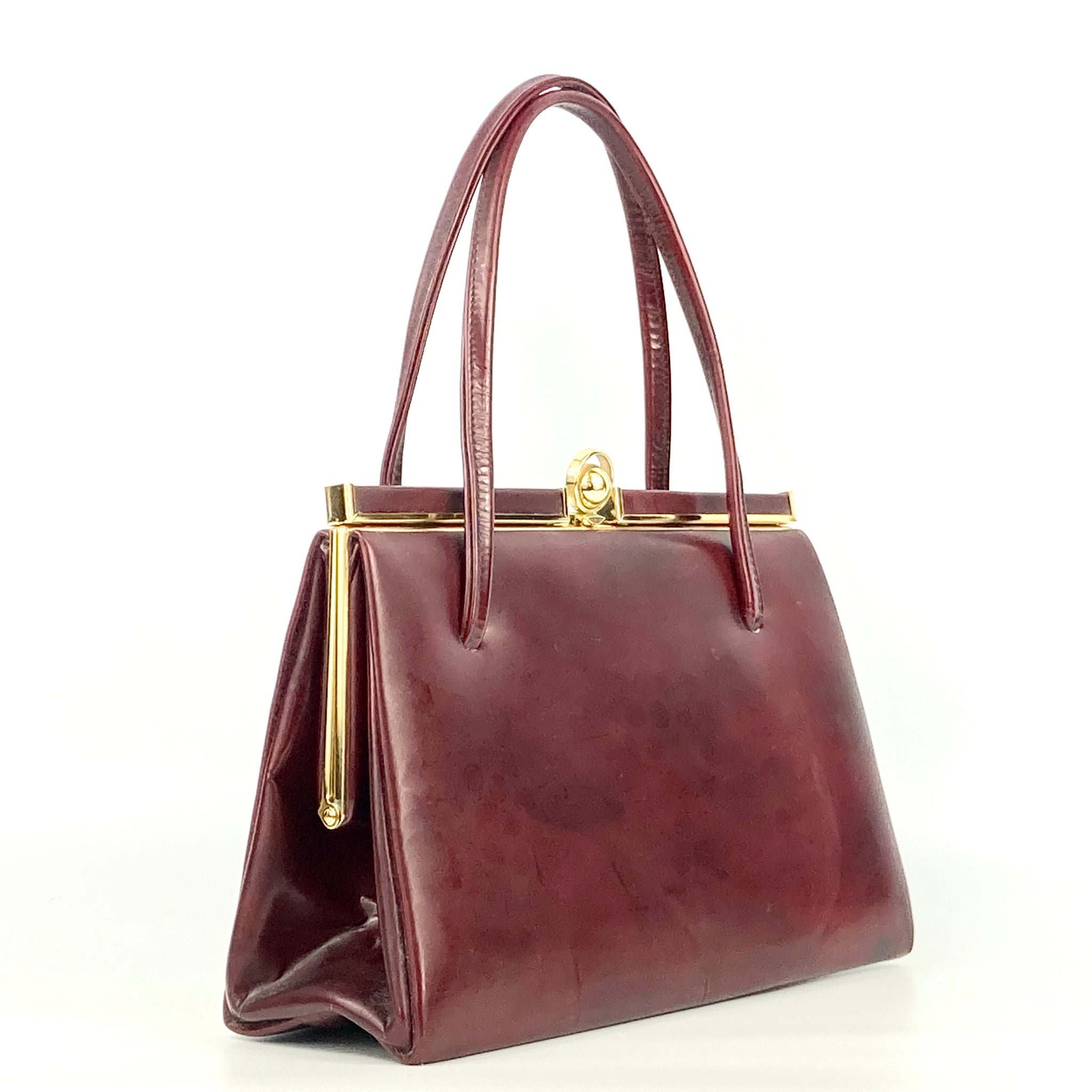The image features a maroon leather handbag, poised upright on a white surface. The bag is illuminated from above, casting distinct shadows underneath, which might include a wooden edge adding a hint of texture. The material of the purse is somewhat reflective and shows variations in color from rich maroon to darker, almost reddish brown hues, with some areas appearing dusty or stained due to light reflections. It has a gold-colored clasp and trim near the top, extending into hinges along the sides. The purse is structured with two sturdy handles arched gracefully over the main body, maintaining their shape. The flat base allows it to stand independently, and while there are no discernible brand markings or external pockets visible in the image, the simplistic design is accentuated by the interplay of light and shadow.